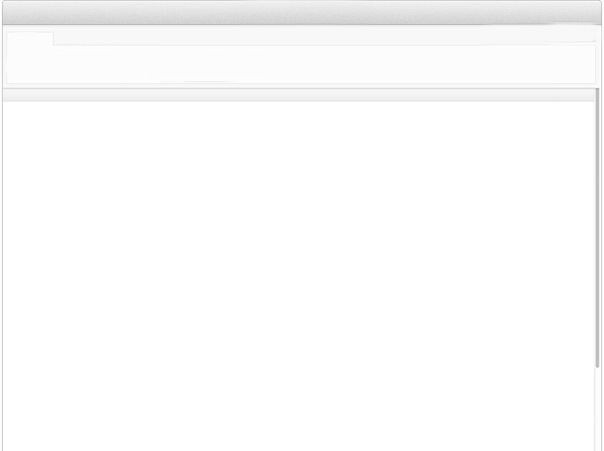The image is a screenshot of a predominantly blank page, marked by its pristine, highly white background with no text or notable features. The page is slightly rectangular and oriented in a landscape layout, approximately measuring 45 by 55 units. 

On the right-hand side, there is a very thin vertical border consisting of gray lines, adjacent to a slightly thicker gray line that doesn’t extend as far down the page. This thicker line might represent a scroll bar for navigation. 

At the top of the image, there is a thin gray bar followed by a section in a lighter shade of gray, which transitions to an even lighter, almost white, rectangular section. This section is slightly irregular, with a slight bump on the left-hand side. Beneath this, another gray line spans horizontally from left to right. The lower portion of the image is entirely white, completing the minimalist and unadorned appearance of the page.